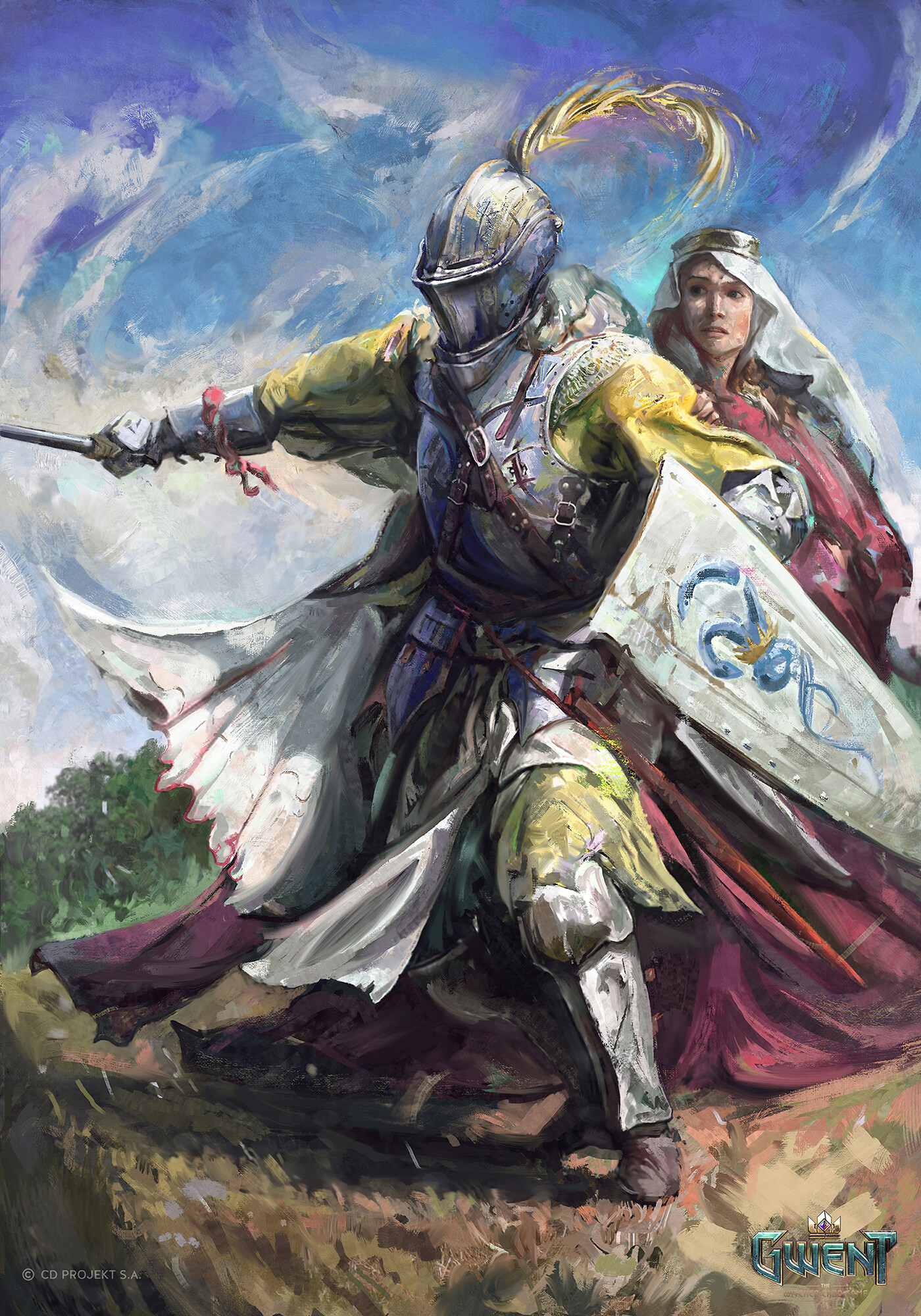The image depicts a dramatic painting of a medieval scene. At its center is a knight in full, shining armor, complete with a metal steel helmet adorned with a yellow plume, a breastplate, and armor extending to his knees and legs. He wields a sword in his right hand and bears a shield with a blue design, possibly featuring a dragon and a snake, in his left. His attire includes a yellow garment under the armor with brown shoes visible.

The knight stands protectively in front of a woman dressed in a flowing pinkish-red gown with a white headdress, suggesting she might be a princess in distress. The woman appears to be seeking refuge behind the knight. The setting is a countryside with a hill adorned with patches of greenery and browns, and in the distance, a sky swirling with blue and white clouds adds drama to the scene.

At the bottom right corner of the painting, there is a signature, possibly reading "GWENT," though it's somewhat unclear, and a watermark crediting "CD Projekt SA" can be found in the bottom left corner. This richly detailed scene captures a moment of valor and protection set against a backdrop of natural beauty.